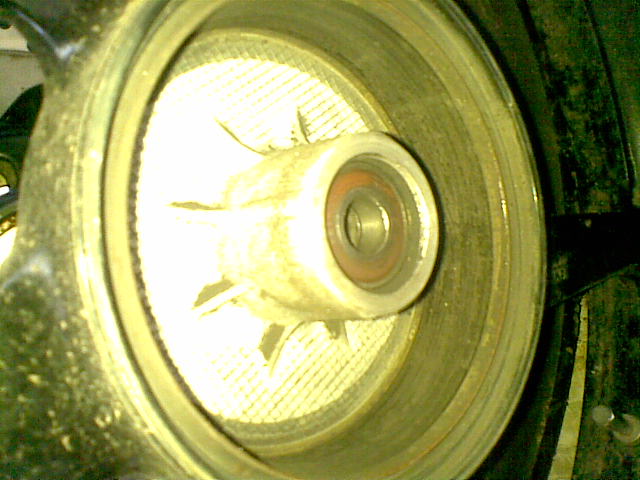This close-up, square image captures a large, circular, metallic object, possibly part of a car's internal mechanism. Dominated by a grayish-brown hue, the object is framed by an outer gold rim that adds a sparkly touch to its appearance. The inner section resembles a glowing spotlight, highlighted by a nearly white hue. At the very center, a rusted washer-like component can be observed. This section protrudes outward, forming a cylindrical shape with a central hole. Surrounding the object, a black area encircles the back, with a greenish-black tint on the right side and a blurry, sparkly gray and gold area on the left. To the left, a partially visible speedometer suggests that this object might be part of a steering column, specifically the hub behind where a steering wheel would typically be mounted. The overall image is slightly blurry, adding to the mysterious, metallic allure of the component depicted.